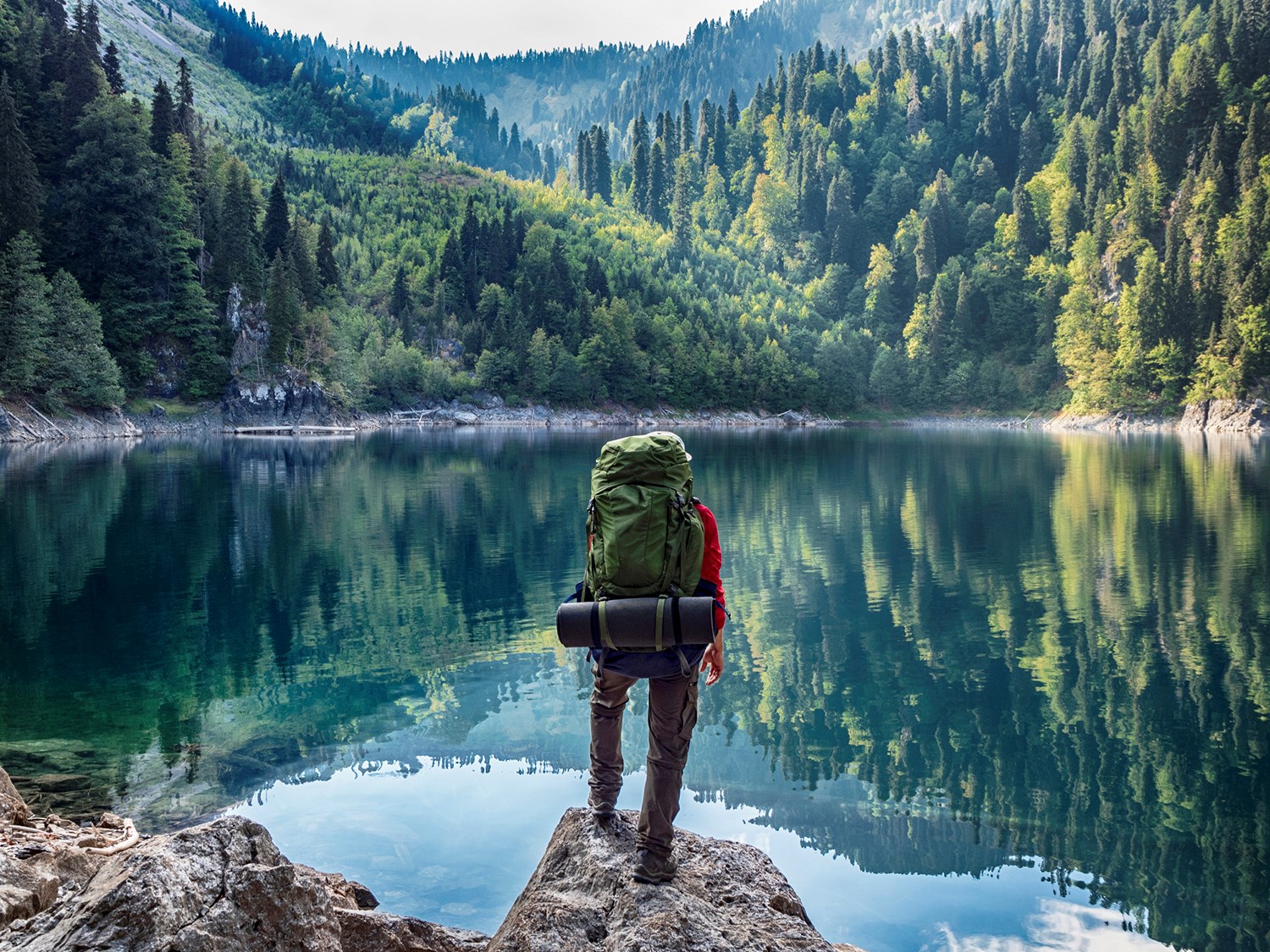This high-quality image captures a serene and picturesque scene of a backpacker standing on a rocky outcrop, overlooking a calm and reflective mountain lake. Clad in a red long-sleeve shirt, gray hiking pants, and boots, the hiker stands with his back to the camera, wearing a green backpack with a rolled-up sleeping pad attached at the bottom. The lake’s glassy surface mirrors the surrounding landscape, showcasing an array of tall, dark green, light green, and medium green pine and fir trees. These trees ascend a steep hill leading up to a mountain peak, creating a beautifully layered and hilly backdrop. The tranquil setting evokes a sense of peaceful solitude, reminiscent of the pristine wilderness found in places like Colorado.